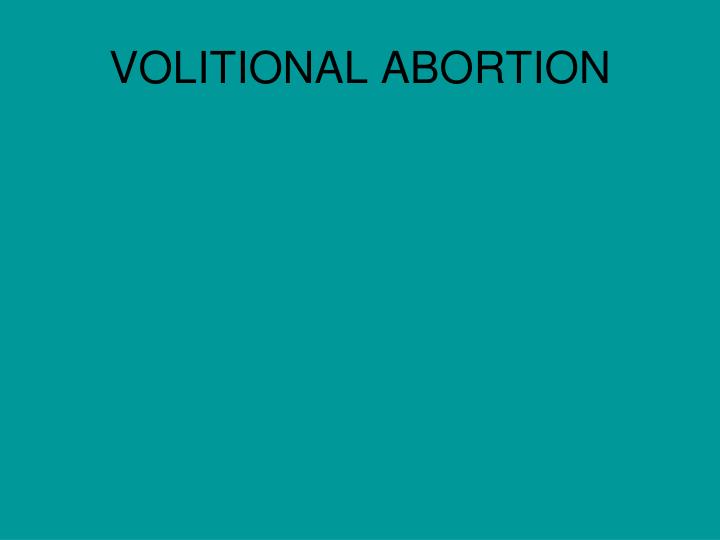The image is a simple, turquoise or teal-colored PowerPoint slide with a clean, blue-green background that evokes the serene hues of a tropical ocean or a cloudless sky. At the very top of the slide, in plain black text, the words "Volitional Abortion" are prominently displayed in all capital letters, appearing as "V-O-L-I-T-I-O-N-A-L  A-B-O-R-T-I-O-N". The text is written in a small, centered font, exhibiting a slight distortion inherent to its style. Aside from this succinct title, the slide is devoid of any other visual elements or text, presenting a minimalist and straightforward design.